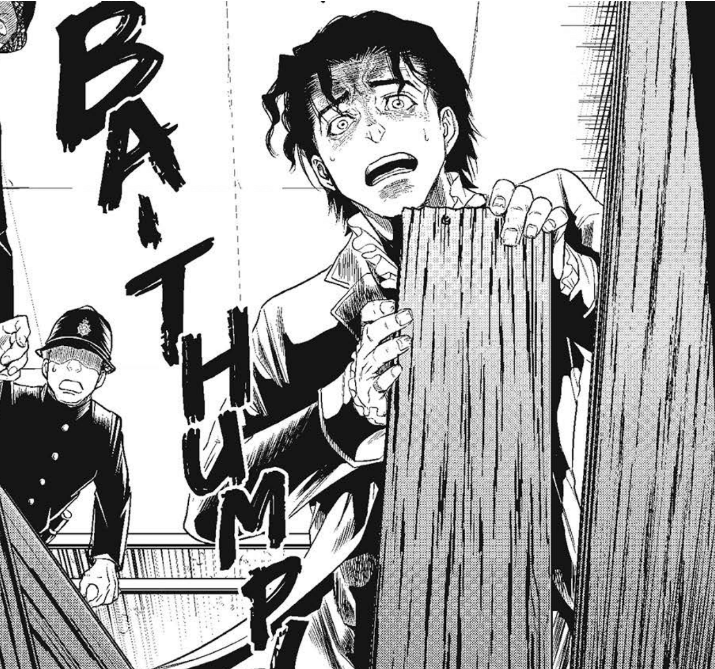In the black and white manga panel titled "Be a Thump," the illustration captures a tense moment featuring two figures. The title is painted vertically on the left side with "B-A" at the top and "T-H-U-M-P" below it. In the foreground stands a man with wavy black hair, his eyes wide with terror and mouth agape. The wrinkling in his eyebrows and forehead highlights his alarmed expression. He dons a fanciful outfit, complete with a blazer, cape, and ruffled collar, and clutches a vertical wooden board with both hands. It appears he is attempting to break through a fence, possibly trying to squeeze through it. In the background, a police officer, wearing a helmet and black uniform adorned with buttons, is partially visible. He too looks worried as he leans into the frame, his body only shown from the waist up. This scene combines old-school American comic elements with a touch of anime style, evoking a sense of vintage urgency and drama.